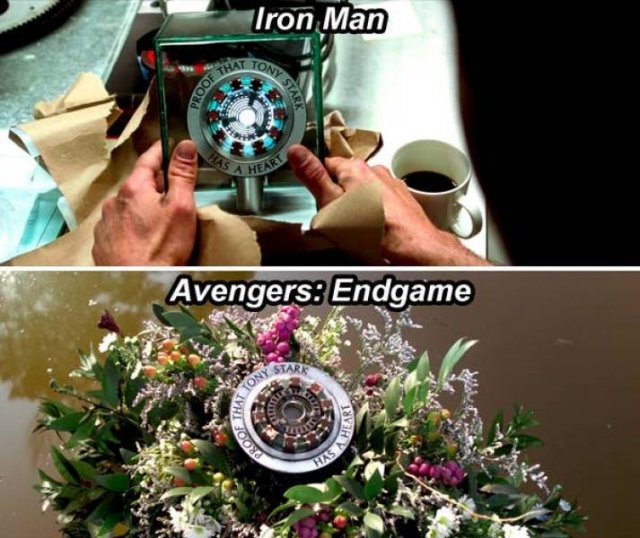The image features two juxtaposed photographs from different scenes in the "Iron Man" and "Avengers: Endgame" movies. The top photograph, an older screenshot from the first "Iron Man" movie, captures a moment where Tony Stark is seated at a table, unwrapping a special gift from Pepper Potts. The gift is a circular LED light trophy inscribed with "Proof that Tony Stark has a heart." The glass encased trophy lies on the table beside torn brown craft paper and a half-filled white coffee mug. The word "Iron Man" is prominently displayed in white text bordered by black imposed over this scene. 

The bottom photograph is a scene from "Avengers: Endgame," the final Avengers movie, and showcases the same trophy now placed amidst a beautiful floral arrangement, likely symbolizing Tony Stark's funeral tribute. This scene reflects the trophy’s transformation from a personal memento into a meaningful commemorative piece. The positioning and colors of both photos highlight a stark but poignant comparison—emphasizing the journey and legacy of Tony Stark's character.